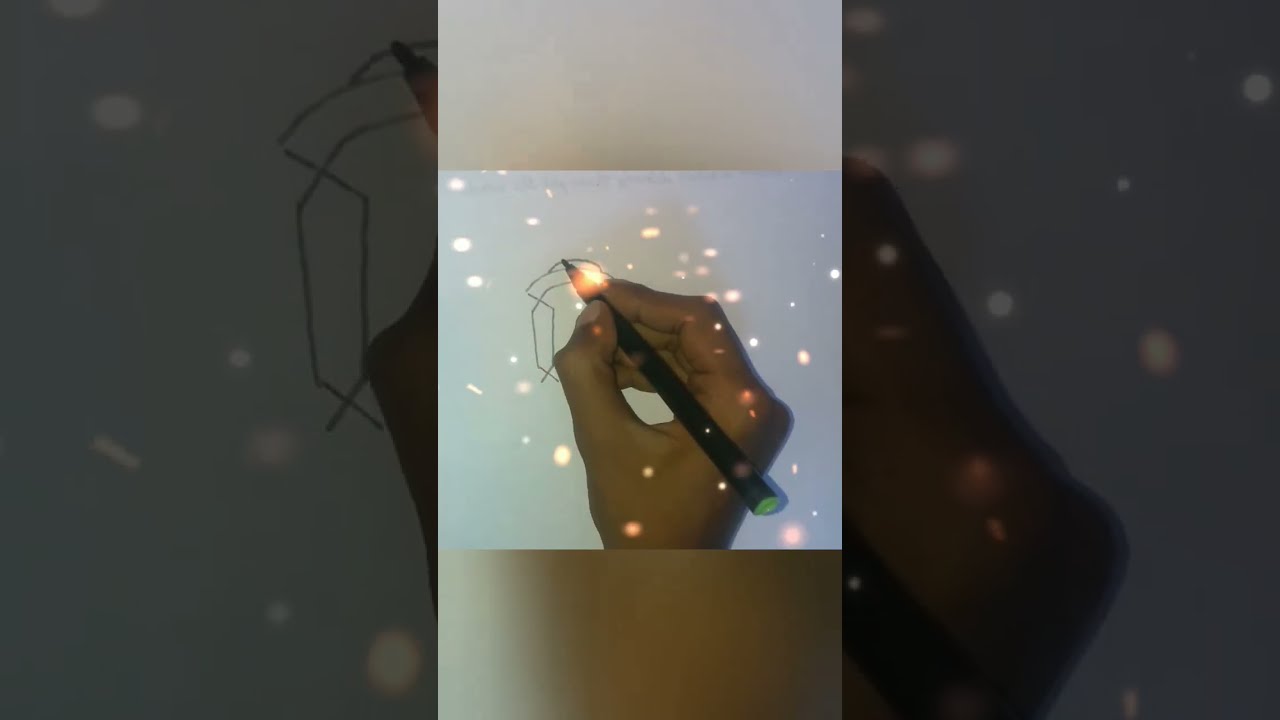The image captures a dark-skinned right hand in the process of drawing on a white piece of paper. The hand holds a black pencil with a green eraser, delicately sketching a few lines that do not yet form a recognizable image. This central scene is encased within a vertical rectangle, and the entire composition is overlaid against a darker, shadowed, and blurred version of the same image, creating a repeating and layered visual effect. The background image is larger and more subdued, emphasizing the lit-up segment in the middle. Overhead lighting casts circular spots of light onto the paper and the hand, adding depth and focus to the drawing activity. A significant shadow from the hand stretches across the scene, highlighting the meticulous moment of the creative process.